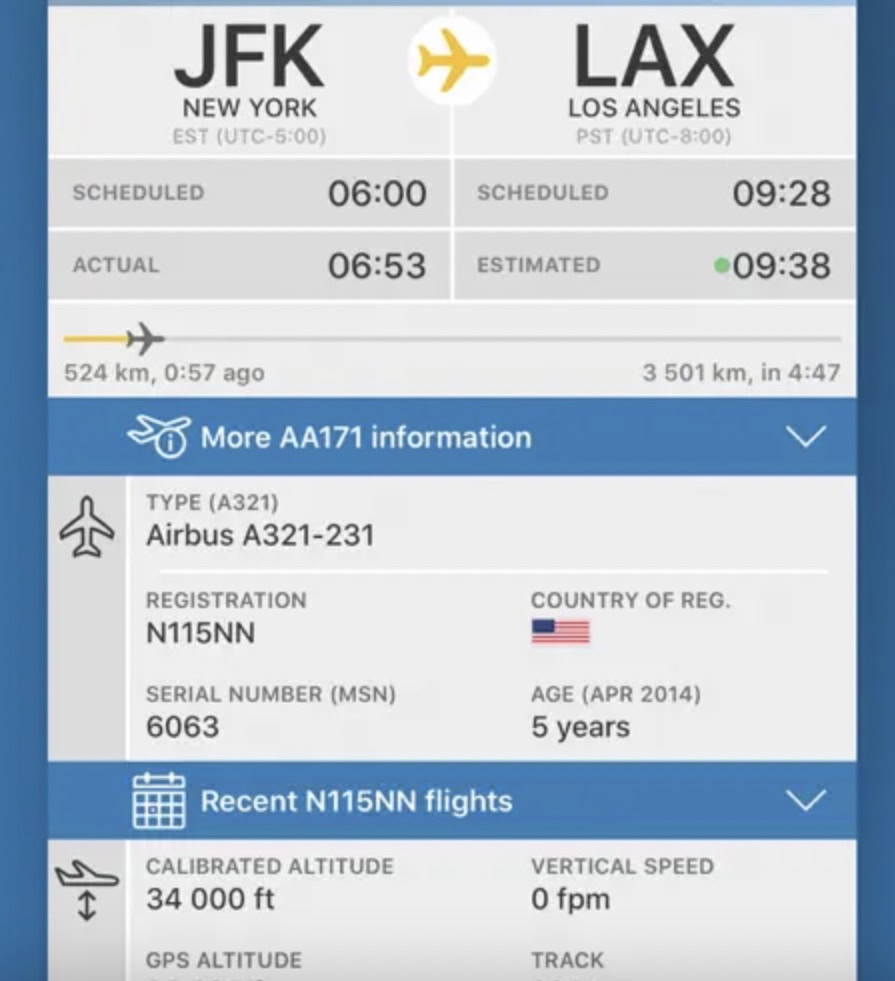This image appears to be a detailed screenshot of someone’s flight itinerary displayed on a computer screen. The layout features a prominent blue vertical rectangle adorned with three distinct gray horizontal boxes. The first gray box at the top indicates the flight's departure and destination, stating "JFK New York" on the left and "LAX Los Angeles" on the right. Between these, there is a small yellow airplane icon enclosed in a white circle moving towards the right. The text underneath displays scheduled and actual departure times: "Scheduled 6:00" and "Actual 6:53." For the arrival at LAX, it shows "Scheduled 9:28" and "Estimated 9:38," indicating a slight delay.

Below this, a horizontal line with a small airplane icon illustrates the flight's current position or progression. The blue area features flight-specific links and information, denoted by a plane symbol and the text "More AA 171 information," accompanied by a downward arrow.

In a subsequent gray box, additional aircraft details are provided. It includes another airplane symbol pointing upward and to the left, with the text specifying the aircraft type as "Airbus A321-231." Further details list the registration number "N115NN," the country of registration marked with an American flag, serial number "6063," and the aircraft's age, "5 years."

Further down in the blue rectangle, under "Recent Flights," it provides more extensive flight data, including "Calibrated 34,000 feet," "Vertical Speed 0 FPM," and terms like "GPS Altitude" and "Track." This comprehensive and meticulously organized screenshot provides a thorough summary of the flight status and aircraft particulars, beneficial for both passengers and aviation enthusiasts.